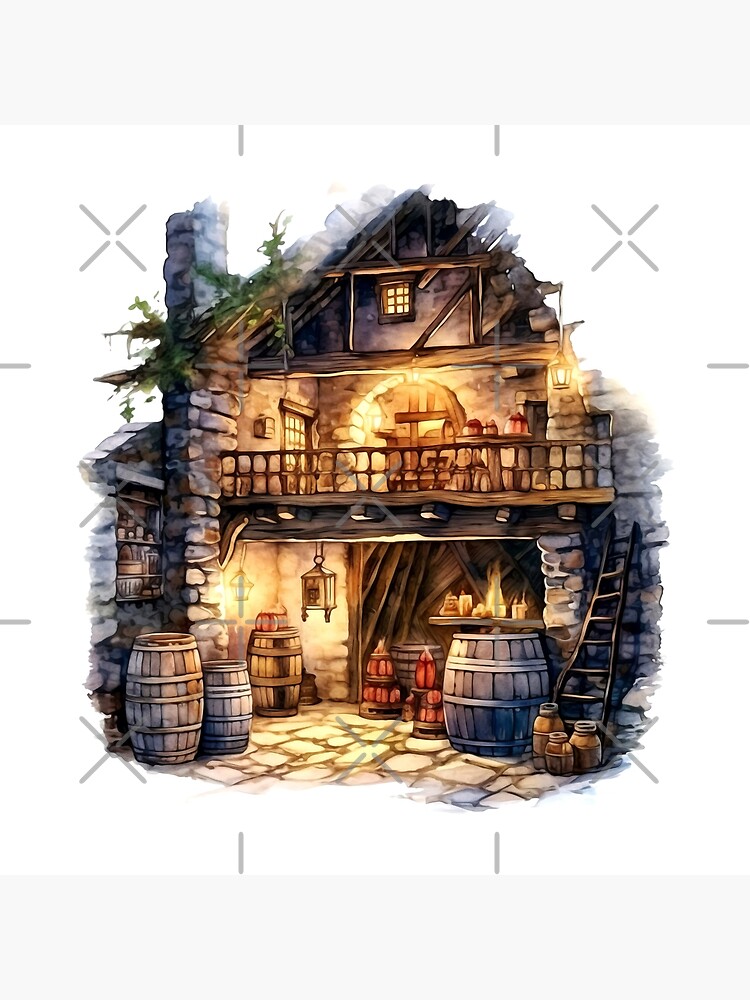This image depicts an intricately detailed illustration of an old-fashioned stone and wooden house, reminiscent of medieval times. The perspective offers an x-ray view into the rustic interior, revealing a multi-level structure rich with historical charm. The exterior showcases stone textures and a stone chimney, while inside, wooden beams and stone floors set the scene. The first level features numerous wood barrels, varying in size and color, alongside jars and crates scattered on the ground. A wooden ladder leans against the wall, leading to the second floor where more barrels, jars, and a wooden railing can be seen. Various lanterns and a light hang from the ceiling and rafters, casting a warm glow. The second floor also has a round opening in the wall, suggesting a cozy hobbit-like entrance, and a rectangular doorway with light spilling from behind it, hinting at further rooms. The third level is represented by just a single window, adding to the quaint and comforting ambiance of the entire dwelling. This detailed illustration might be a design concept, potentially for sale, and exudes a sense of nostalgia and comfort, capturing the essence of a bygone era.